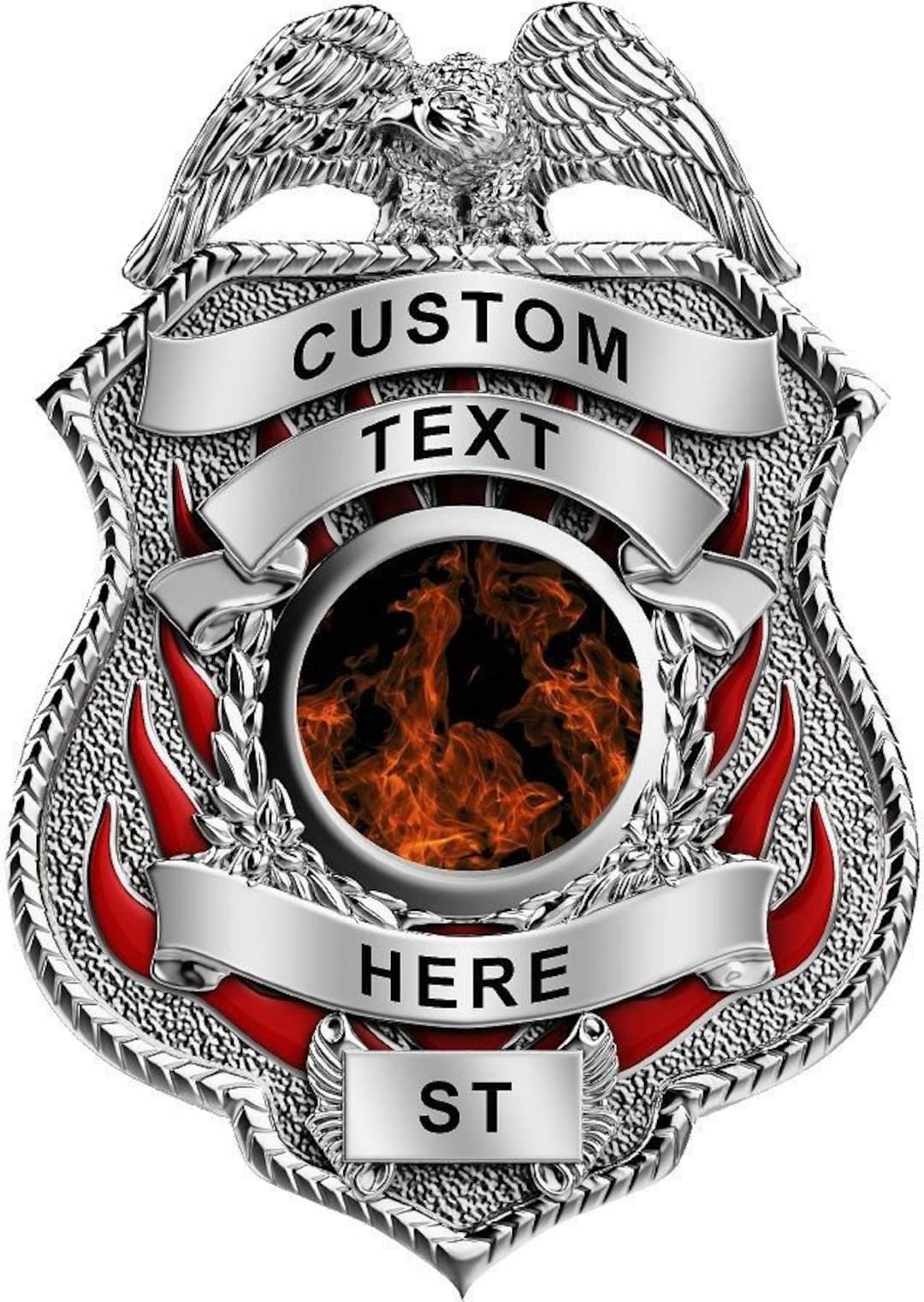This image depicts a computer-generated, enlarged silver badge against a white background. At the top of the badge, there's a detailed engraving of an eagle perched and looking to the side. Below the eagle are two banners: the top one reading "Custom" and the one beneath it saying "Text." At the center of the badge, there's a silver circle adorned with what appears to be a holographic or 3D depiction of flames. Surrounding this central circle is a laurel wreath crafted in silver. Below the flames, a banner states "Here," followed by a silver rectangle displaying the letters "S.T." Red enameled flames embellish the lower part of the badge, extending upwards around the central circle and beneath the top banners. The badge appears to be part of a customizable badge maker or manufacturer.